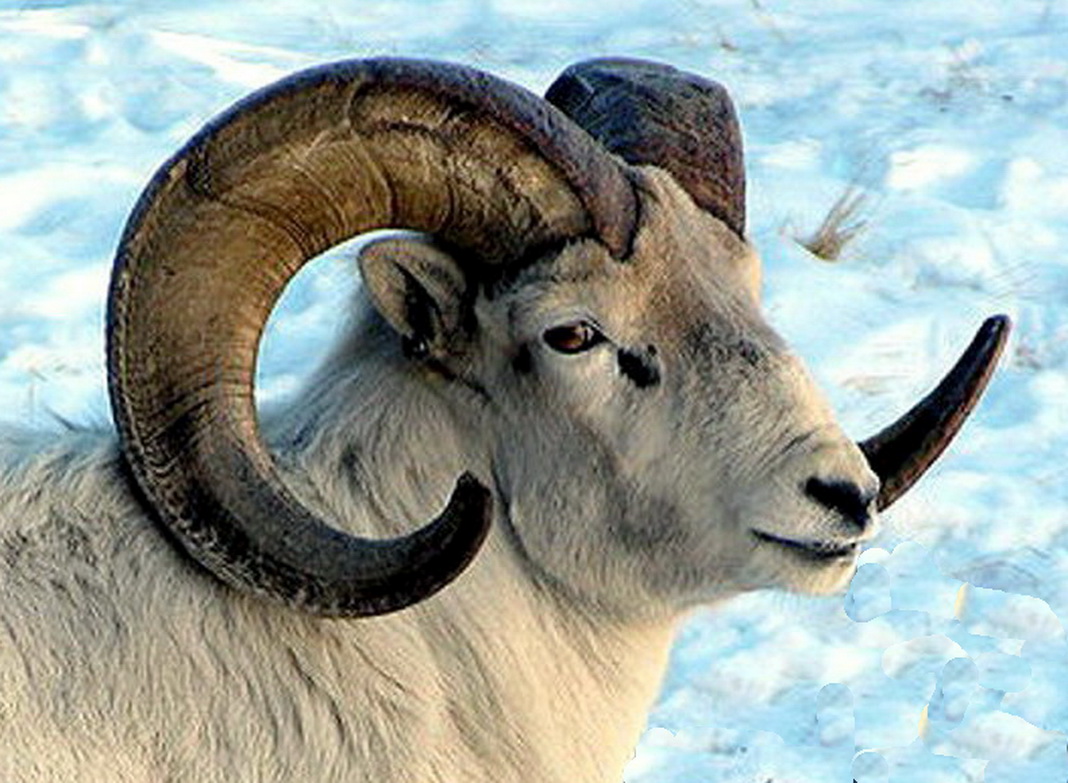The image is a stunning, high-quality, close-up photograph of a longhorn sheep, or ram, taken in a snowy landscape. The background is predominantly white with a glacial blue tint, perhaps due to the way the light is hitting the thick snow. Amidst the snow, there is a solitary tuft of brownish vegetation peeking through.

The ram is captured in its right profile, from about halfway down its back forward. Its enormous, curving horns, resembling layered sandstone in texture, are brown with black tips, forming a majestic 'C' shape on the sides of its head. The animal's coat is a cream white with some tan, and it's adorned with various black markings: prominent black scent glands under the eyes, a black-tipped nose, and dark accents around its eyes, which are a light brown color. The ram's small, rounded ears lay back against its head. One of its most striking features is its enormous horns, which enhance its regal appearance. This magnificent creature stands out vividly against the snowy backdrop.